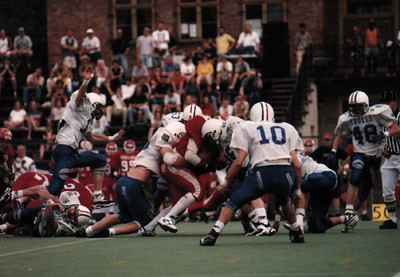This photo captures an intense moment in a high school football game. The game is taking place on a vibrant green turf field, where a player in a red uniform is fiercely running with the football, while players in white jerseys with blue numbers and dark blue pants are attempting to tackle him. The red team is dressed in all red with white stripes down their pants, and the white team's numbers "10" and "48" are visible. In the background, a crowd of older spectators watches the game from the stands near a red brick building with black stairs and banisters. The scene is packed with action as the red team runner battles to advance the ball, illustrating the determination and competitive spirit of high school football.